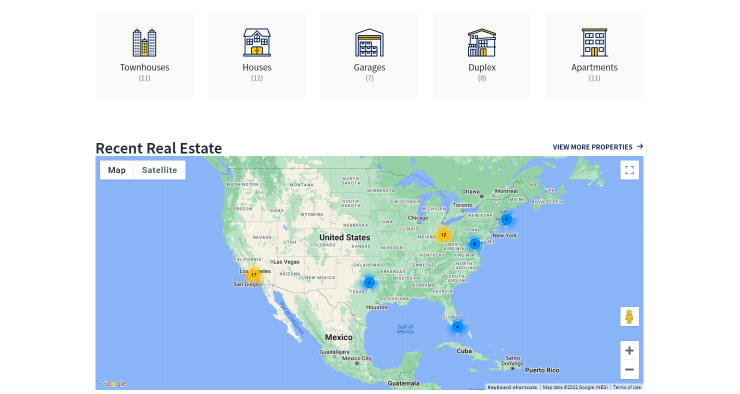This image is sourced from a real estate website and is meticulously structured to present various property options. At the top of the image, there are five selection boxes displayed horizontally. Each box is light gray and features a black font label along with a corresponding icon highlighted in blue and yellow. Below each label, there are numerical indicators showing the quantity of listings available. The categories from left to right are as follows: Townhouses, Houses, Garages, Duplex, and Apartments.

The background of the website outside of these boxes is white, providing a clean and uncluttered look. Directly underneath these boxes, the site displays a Google Map of the United States. Above this map, a heading reads "Recent Real Estate" in black font. On the right side, above the map, there is a call to action that says "View More Properties" in navy text accompanied by a right-pointing arrow button.

The map is specifically centered to cover the US and parts of Mexico, showing the distribution of real estate listings using colored circles. These circles are color-coded based on the categories they represent: yellow and blue. For instance, around the Los Angeles area, there is a prominent yellow circle with the number 17. In contrast, Texas has a blue circle with the number 4, and similar blue circles with the number 4 can be found in Florida, around New York, and in the Mid-Atlantic region. Additionally, there is another yellow circle located in the Midwest.

Overall, the image provides an organized and visually clear overview of real estate options available across the United States, making it user-friendly and informative.